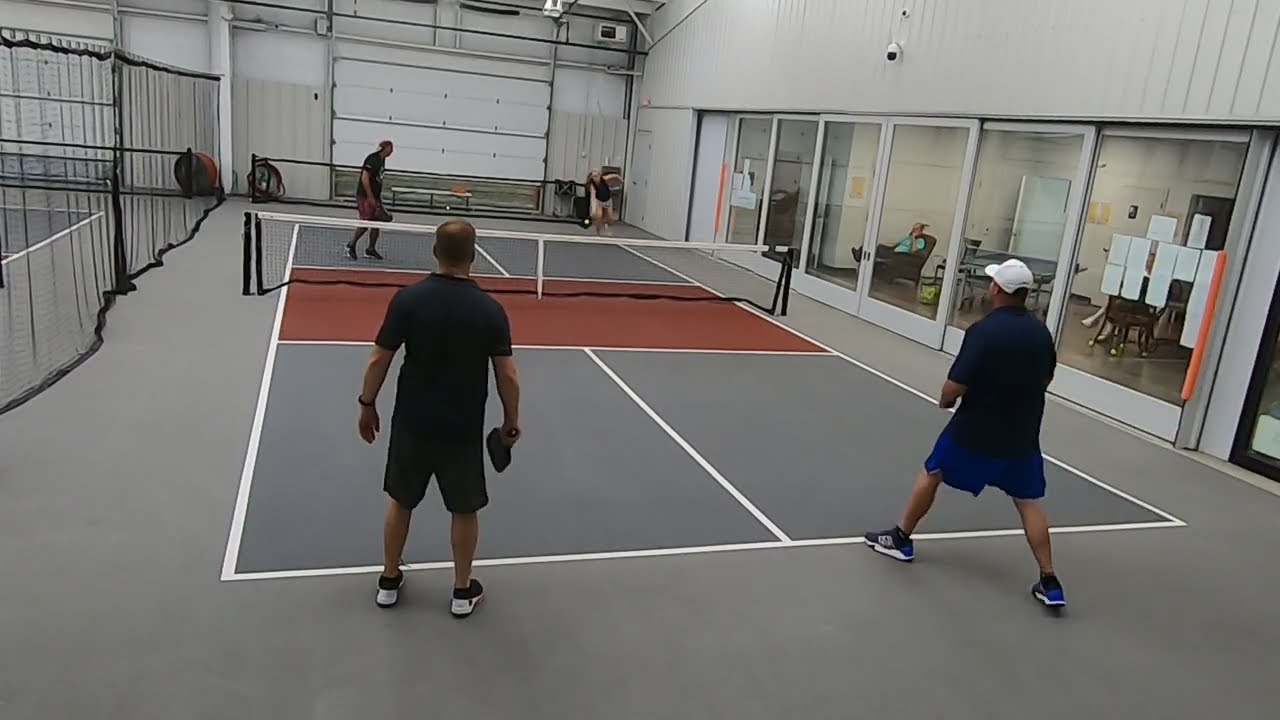The image captures an indoor badminton court surrounded by a gray flat surface, delineated by distinct white lines marking various sections. The court is bustling with activity, featuring a two-on-two game with four players. The player on the far right stands out in a blue shirt and shorts, black and blue shoes, and a white cap. The building itself has an industrial aesthetic, characterized by metallic walls and a large metal rolling door on the far side.

On the left, a collapsible fabric fence separates this court from an identical adjacent one. The right side of the image reveals multiple glass rolling doors, behind which people are seated in armchairs, spectating the game. The arena's color palette is dominated by shades of gray, blue, black, and white, intensifying its modern, utilitarian feel.

In addition to the primary court, there appears to be a small area that might contain a ping-pong table or similar recreational equipment, enhancing the space's multifunctional nature. The overall scene is set in a recreational sports complex, emphasizing the spirited, competitive energy of the ongoing badminton match.